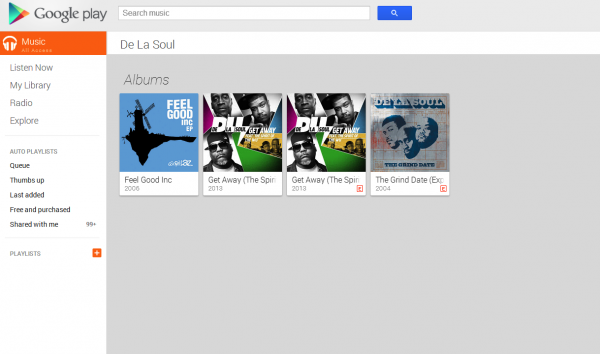The image depicts a Google Play webpage focused on music. At the top, there's a search box with a magnifying glass icon beside it. Below the search box is an orange tab labeled "Music," which features an icon of a pair of headphones. To the right of this tab, "De La Soul" is displayed.

Below the "De La Soul" header, there's a section labeled "Albums" with several entries listed:
1. "Feel Good Inc." - 2006
2. "Get Away" - 2012
3. "Get Away Again" - 2013
4. "The Grind Date" - 2004

On the right side of the page, there are additional tabs for various functionalities: "Listen Now," "My Library," "Radio," and "Explore." Further down, there are options labeled "Thumbs Up," "Last Added," "Free and Purchased," "Shared With Me," and a "Playlists" section with a plus sign next to it for adding new playlists.

Overall, the webpage serves as an interface for browsing and managing music, with a specific focus on albums by De La Soul.